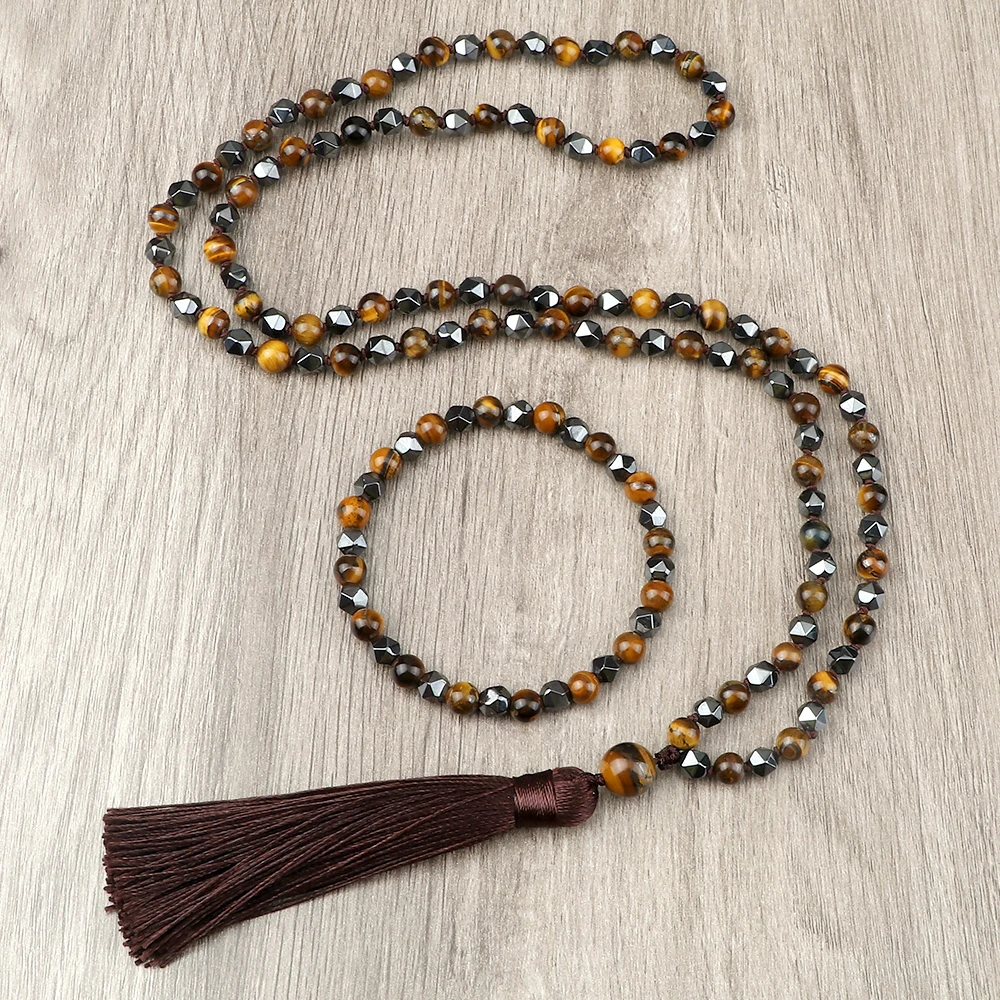The image showcases a beaded necklace and bracelet arranged on an unfinished, rustic wooden table, which exhibits a light brown to dark grain and a rough texture suggestive of potential splinters. The necklace, featuring a consistent pattern of shiny amber-colored beads alternating with geometric, silver-like beads that resemble facets of a diamond, gracefully circles and curves around the bracelet placed at the center of the image. Each bead is meticulously patterned in a sequence: amber, metal, amber, metal. This theme carries through to the bracelet. At the end of the necklace hangs a lush tassel, composed of brownish-red threads with hints of maroon and light pink, adding a touch of elegance and texture to the composition. The overall setting appears akin to a styled product image, highlighting the detailed craft of the jewelry against the rustic charm of the wooden tabletop.